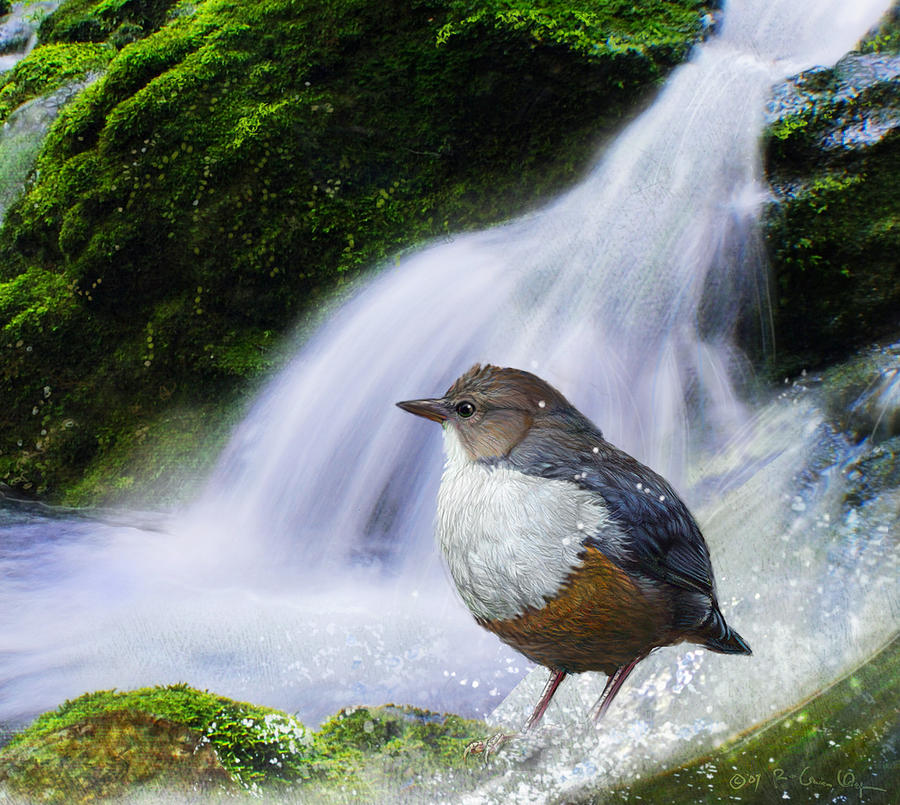This is a detailed painting of a vibrant natural setting centered around a picturesque waterfall that cascades from the top right and flows down to the bottom middle of the image, interwoven with streams winding through clusters of lush, green moss. Dominating the foreground is a round-bodied bird, characterized by its brown head, small beak, and silver-blue feathers on its back. The bird's neck and chest are mostly white, transitioning to an orange underbelly and supported by its long, skinny legs. Its detailed brown eyes seem to watch over the serene environment. The background is lush with greenery, including trees and leaves, enveloping the scene in shades of vibrant and lighter green, adding to the sense of a rich, natural habitat. This artwork, devoid of any textual elements, beautifully captures the tranquil essence of a secluded woodland area.